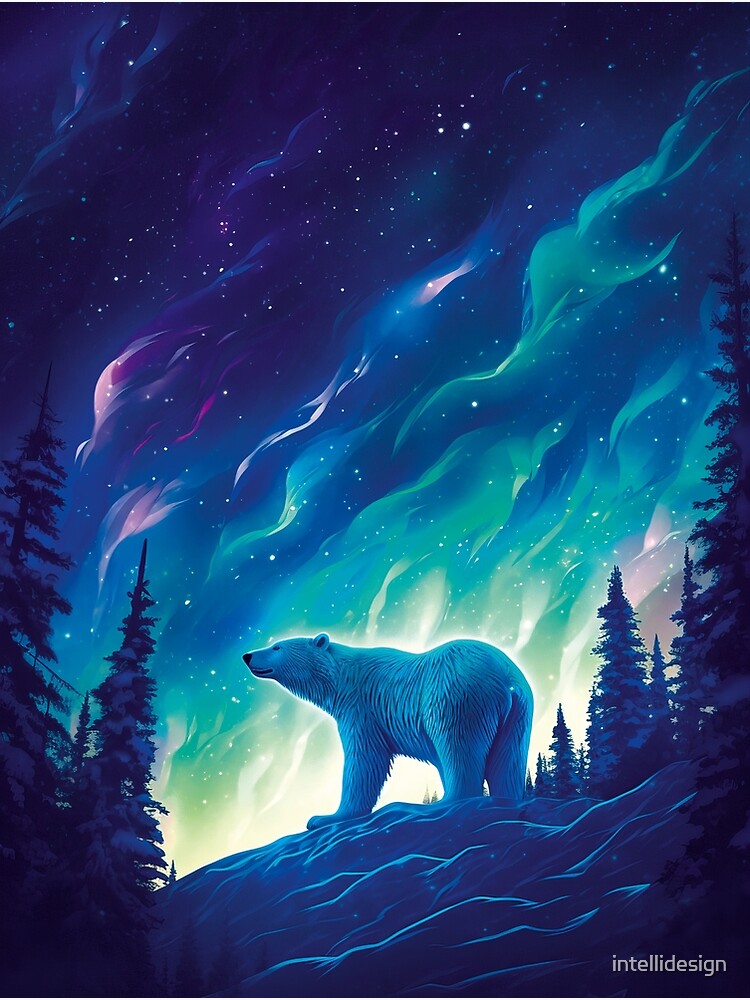This is a digital illustration of a polar bear in a stunningly rich blue and purplish-blue palette with some touches of green and white. Set against a night sky, the scene is dominated by a mesmerizing aurora borealis that streaks across the sky in vibrant hues of white, green, and purple. The sky also features an array of white stars that add to the ethereal atmosphere. In the center towards the bottom, the polar bear stands on a blue, snowy surface, facing left, its fur tinged with blue under the glow of the night sky. On either side of the bear are tall, slender pine trees, dusted with snow and silhouetted against the luminous backdrop. The image exudes a sense of serene illumination, with bright white light emanating from behind the polar bear. The ground beneath the bear is a blend of blue and white, mimicking the overall cool tone of the artwork. At the bottom right corner, "IntelliDesign" is written in crisp white letters, grounding the image with a touch of text.